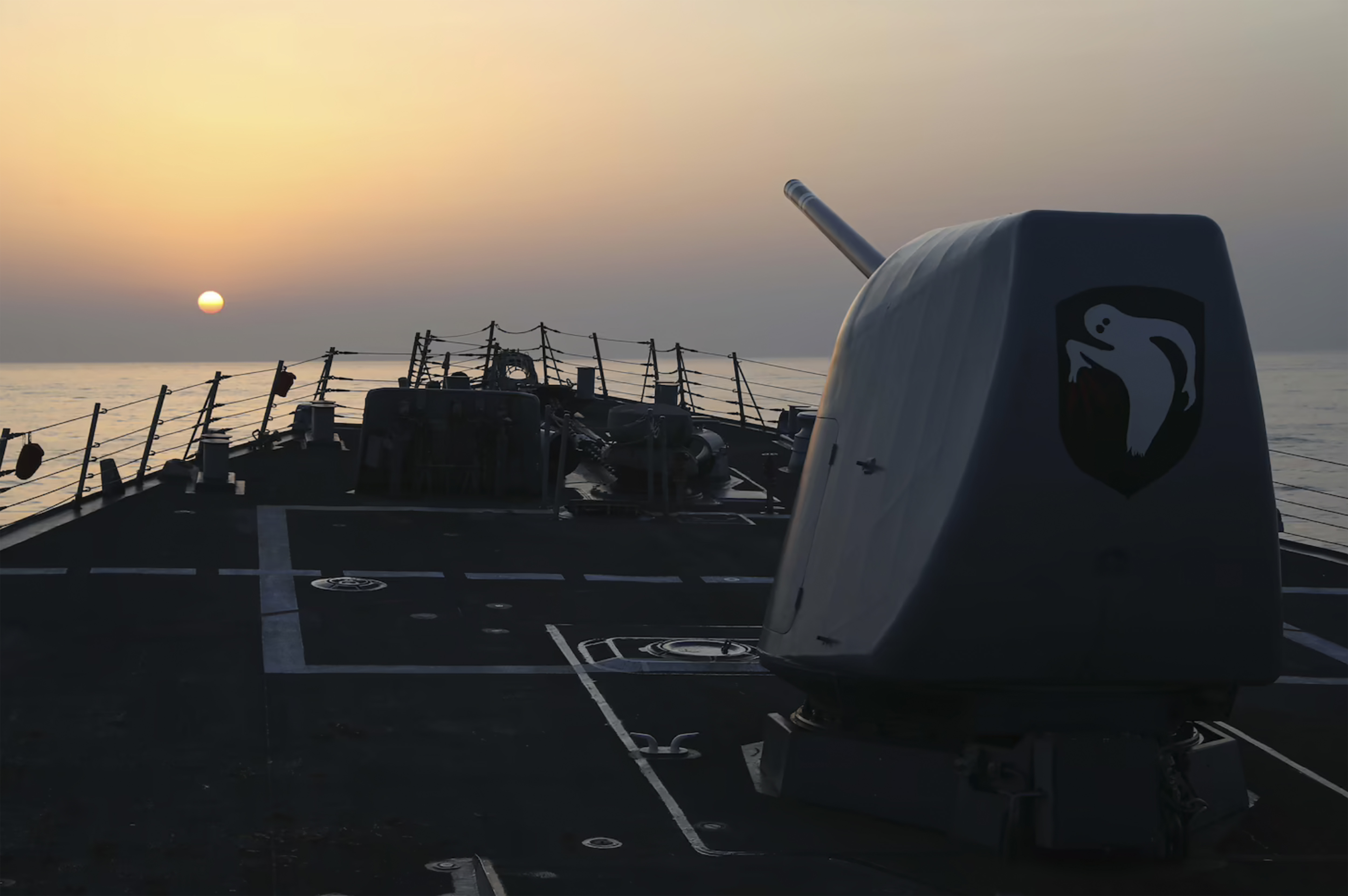The photograph captures the bow of a formidable military battleship, viewed from the midsection looking forward. Dominating the scene is a massive gray gun or missile launcher situated on the right-hand side, its barrel held by a mechanism adorned with a black shield symbol featuring a haunting white ghost. The deck of the ship, a dark gray, stretches out towards the front, fenced by a wire railing that ensures safety along the top edges of the ship. Numerous sections and pieces of metal equipment are scattered across the bow, contributing to the complex nature of the vessel. Surrounding the ship is a landscape of calm, silver water that extends to a flat horizon. The sky above transitions from a dusky gray near the horizon to a lighter yellowish-orange as it ascends. The setting sun is visible in the left of the image, adding a circular glow to the muted colors of the sky, creating a serene yet powerful scene.